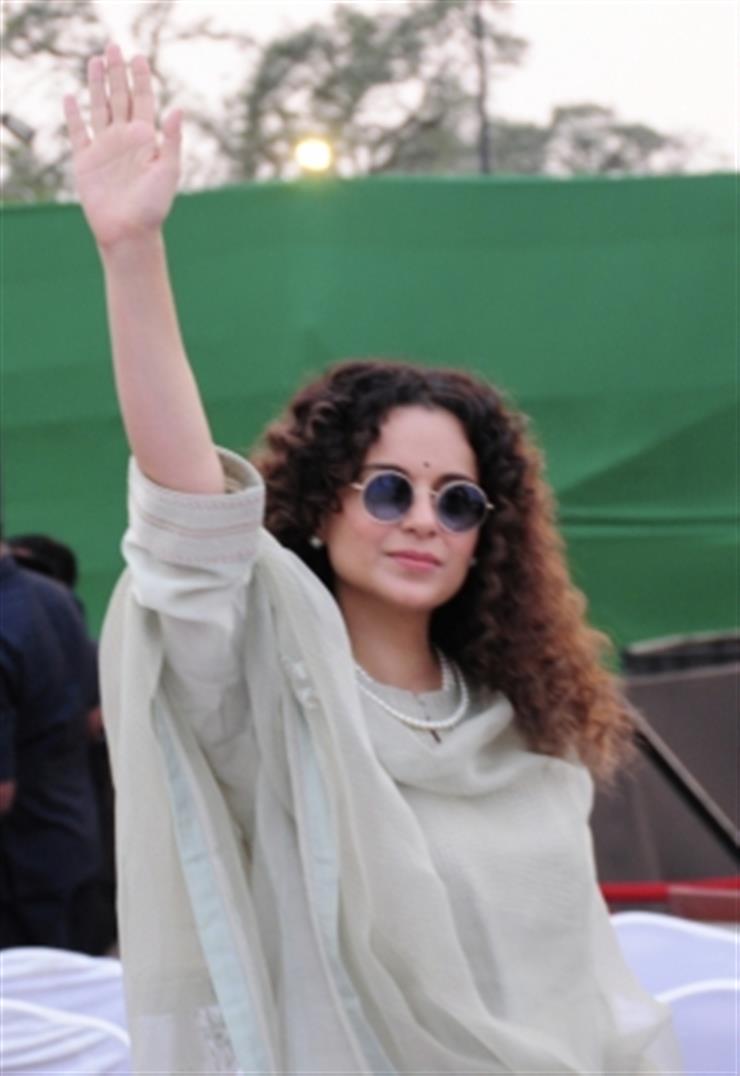In this detailed outdoor photograph, the actress Kangana Ranaut is featured prominently from her face down to her upper body. She dons a loose, flowy gray chiffon outfit that seems to be layered, with sleeves elegantly falling down her arms, complemented by a matching shawl that drapes down. Kangana, who has a pale complexion and a square jaw, accessorizes with a circular necklace and round sunglasses shading her eyes. Her poofy, curly brown hair cascades below her shoulders, encapsulating her ethereal appearance.

Kangana stands poised with one arm raised in the air, as if waving or greeting someone, her closed mouth adding a touch of serenity to her demeanor. The background reveals a green fence slightly visible along with partial glimpses of a couple of other individuals. Beyond the fence, the scene melds into the natural landscape, with the tops of trees silhouetted against a bright yellow sun. The sky appears predominantly white, further accentuating the silhouetted black trees, creating a tranquil yet dynamic backdrop for the photograph.